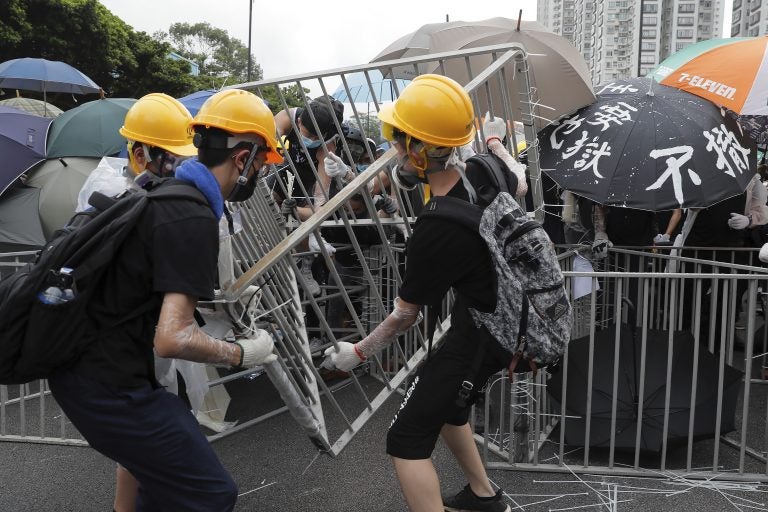In this image, we see a scene of a protest with three individuals lifting a metal barrier typically used for crowd control. These individuals, dressed in all black with orange hard hats and gas masks, are holding the triangular-shaped barrier while wearing gloves and backpacks. The person on the right has black shoes and a gray backpack. In the background, multiple umbrellas in shades of gray and blue, some inscribed with Asian characters—likely Japanese—are visible, suggesting their use for protection. To the left, a series of trees line the top left corner, and a skyscraper rises on the right side, framing the scene with a clear sky above. Scattered throughout the ground are zip ties, hinting at the tension and potential for violence. Moreover, it appears that people are trying to maneuver over the railing, indicating a strike or an escalating altercation where the barrier may be employed to keep the crowd at bay.